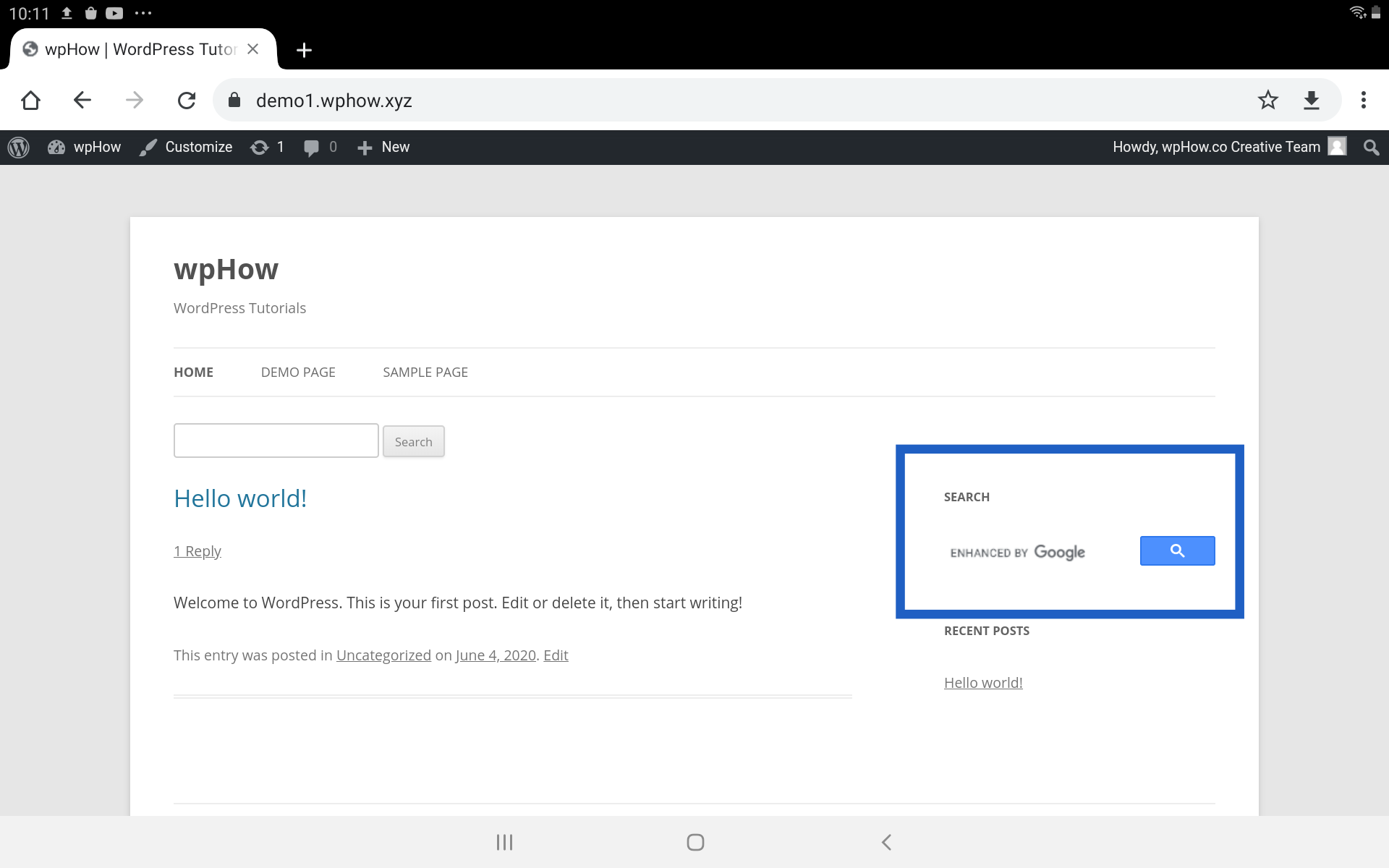This is a detailed screenshot of a website displayed on a tablet running a web browser. At the top of the tablet screen, a black status bar is visible, showcasing the device's time, "10:11," in white font. Adjacent to the time, on the right side of the status bar, there are three small white icons, one of which is recognizable as the YouTube icon.

Directly beneath the status bar, a web browser tab is open with the title "WPHow WordPress," and a globe icon sits to the left of the tab title. Below the tab, the browser's address bar displays the website URL: "demo1.wphow.xyz." To the immediate left of the address bar are several navigation icons including a refresh icon, a left arrow, a right arrow, and a home icon. On the right side of the address bar are a five-pointed star icon and a download icon, represented by an arrow pointing down to a line.

The main content of the webpage is displayed below the address bar on a gray background, with a central white square. At the top of this white square is the heading "WPHow WordPress Tunnel Tutorials" in bold text. Below this heading are navigation links labeled "Home," "Demo Page," and "Sample Page," with "Home" currently selected.